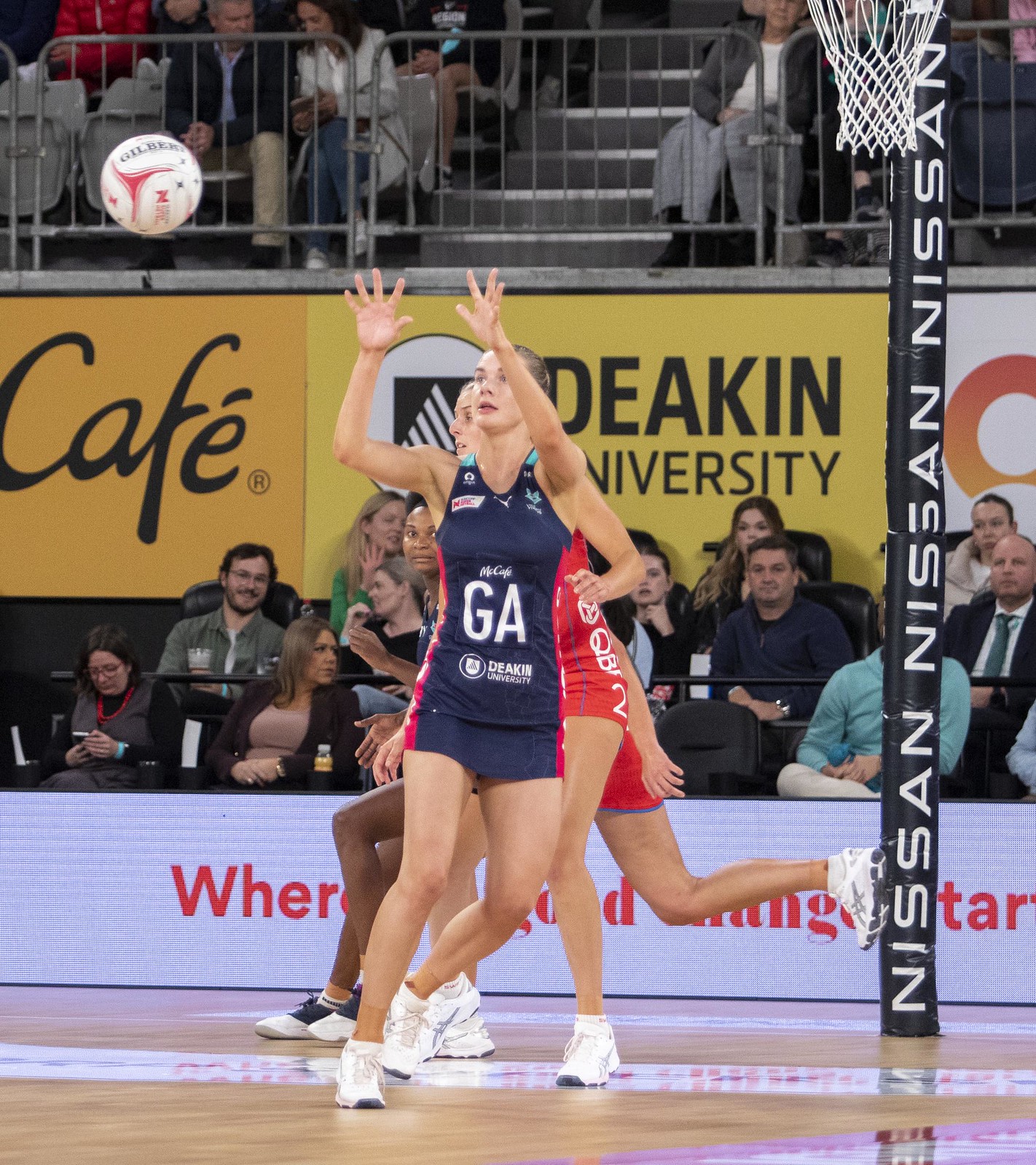This indoor action photograph captures an intense moment during a girls' volleyball match, set within a rectangular gymnasium. The scene centers on a college-aged woman of Caucasian descent in a blue uniform, positioned in the foreground with her arms raised, preparing to receive a volleyball descending from the upper left. The ball hints at imminent action, possibly a pass or a spike. Surrounding her, a tangle of athletes, including one in a red uniform, likely from the opposing team, suggest competitive play, while another teammate in blue stands nearby. The backdrop features two tiers of bleachers with spectators, some engaged with their phones and others chatting, indicating a somewhat relaxed audience. Advertising banners for Deakin University and a cafe line the space between the bleachers. Notably, a basketball hoop adorned with a Nissan-branded protective wrap can be seen to the right, further enriching the gymnasium's setting. The court floor is a light tan wood, adding to the traditional sports environment.